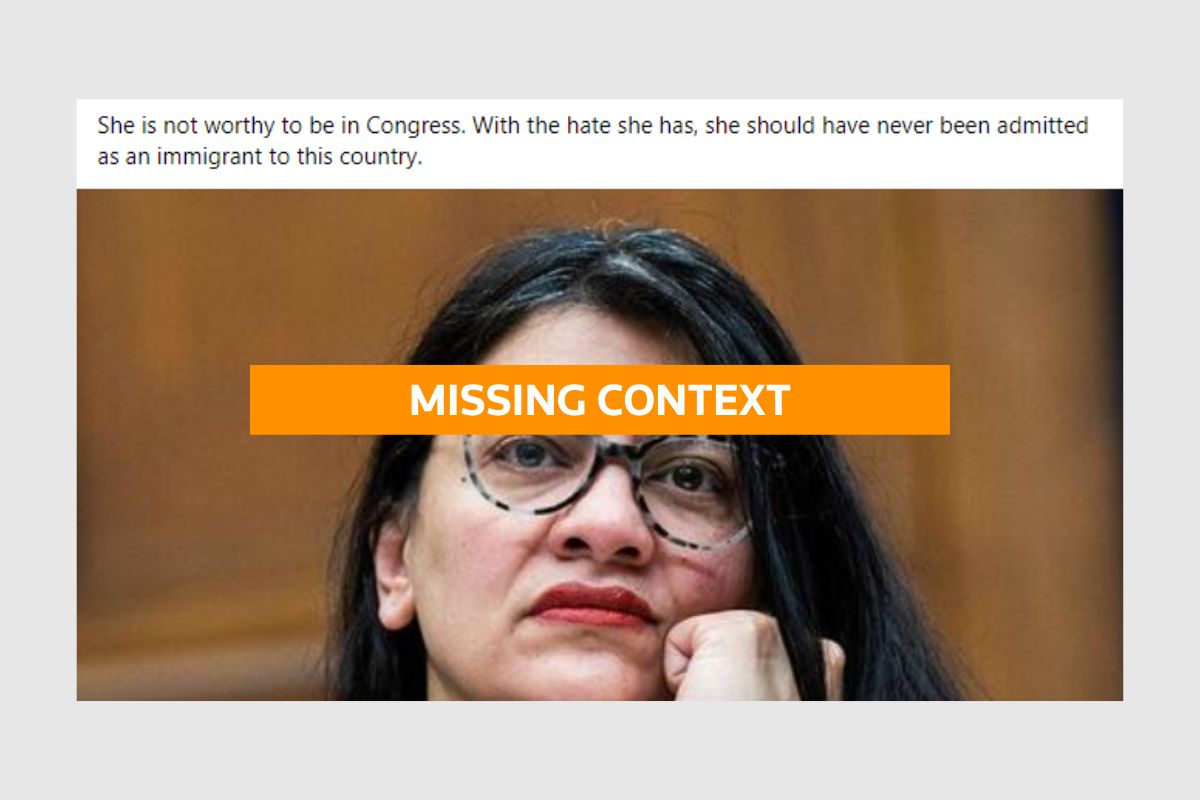The image features a photograph of a woman with distinct characteristics, set against a light to medium gray background. At the top of the image, there is a white banner with black text that reads: "She is not worthy to be in Congress. With the hate she has, she should have never been admitted as an immigrant to this country." Below this, the main photograph captures a woman with silvery black hair, styled with a middle part and slightly more volume on the right side (her left). Her hair includes bangs and a section that is tucked behind her ear, with a lock of hair draping over her fist, which rests under her left cheek. She wears zebra-striped, or possibly spotted, glasses and has bright red lips. Overlaying the photograph, just above her eyes, there is a bright orange rectangle that occupies the central two-thirds of the frame horizontally, containing white text that states: "Missing Context." The background behind the woman in the photograph is a medium reddish-brown, deliberately blurred to focus attention on her.